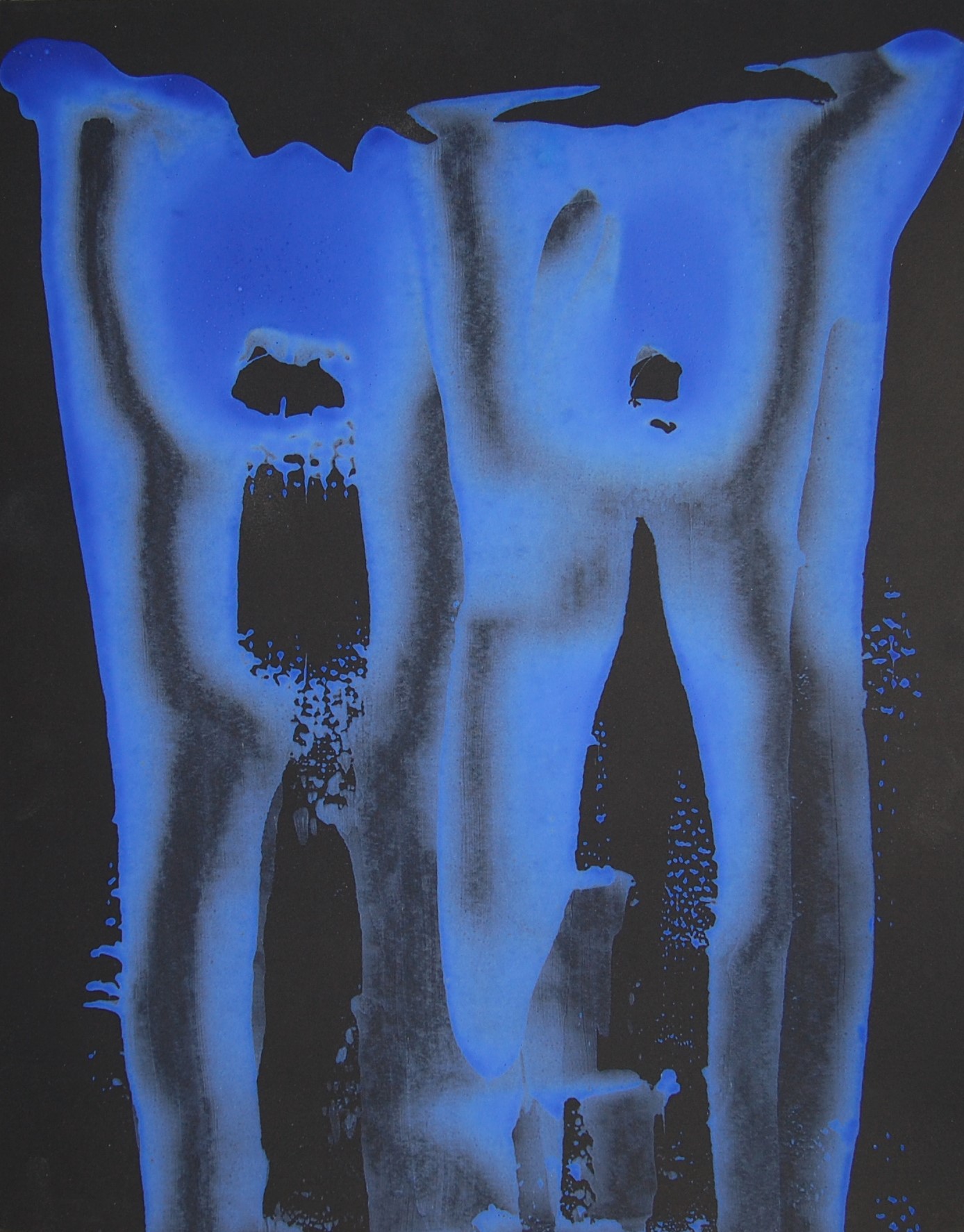This image features an abstract, experimental painting set against a completely black background. The primary color present in the painting is a bright blue, with varying lighter shades that seem to blend into the dark backdrop. At the center of the image, two large blue shapes dominate the composition. These shapes are ambiguous, resembling either two legs standing next to each other or two torsos with legs, suggesting human forms. Each shape has a black line running down its center, with black circles in the torso-like areas. There is also a splatter effect where the paint seems to blur, particularly where the two shapes touch in the middle. Though interpretations vary, the painting evokes the sense of an x-ray or a pair of faces, lending to its modern, abstract style. No text is visible, and additional colors like tan, brown, and gray subtly blend into the artwork, enhancing its intricate and experimental nature.